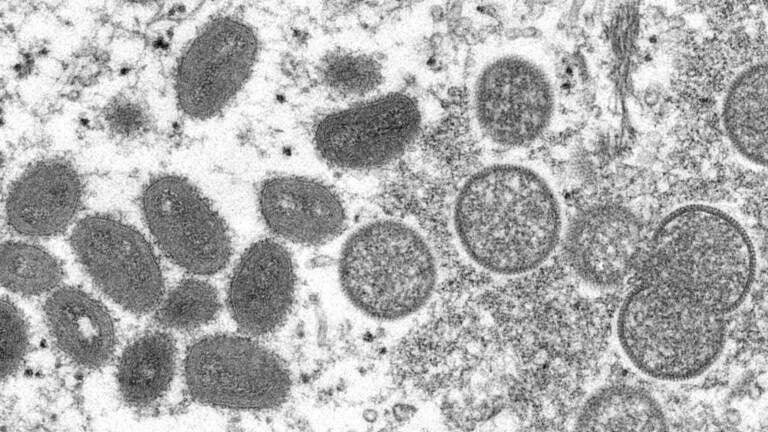This black-and-white microscope image reveals a scene teeming with various microscopic organisms. On the right side of the predominantly white background, several circular cells, approximately five or six, stand out. Each of these circular entities has outer edges adorned with small, spike-like protrusions, resembling the rim of a wheel. Their interiors display a darker, speckled pattern of black and white. Some of these right-hand cells feature a distinct white area, potentially indicating a nucleus.

On the left side of the image, the cells differ significantly in shape and shading. These cells are more oval or kidney-shaped and considerably darker, almost black, interspersed with white speckles. The contrast in shapes and shading patterns between the two groups of cells is notable. The image background is sparsely dotted with black blotches and gray fading, possibly representing dust, food particles, or algae on the microscope slide. Despite the lack of context regarding the time of day the image was taken or the specific type of cells, the detailed contrast and diversity of the cell shapes create a striking depiction of microscopic life.